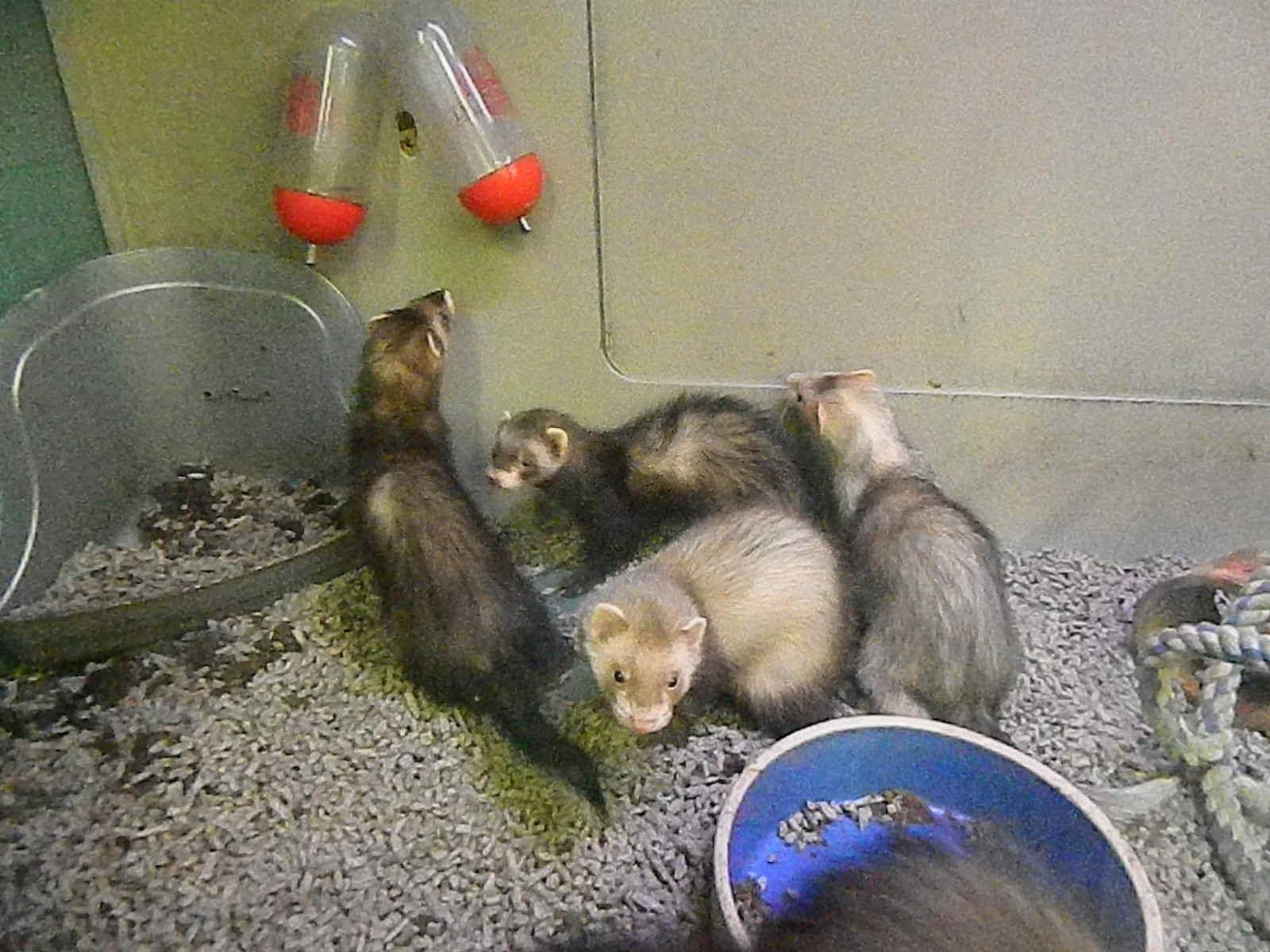The image depicts the interior of a ferret enclosure, housing four small ferrets, one of which is slightly wider than the others. The floor is scattered with wooden pellets, and a blue food bowl with some pellets sits in the bottom right corner. Just beyond the bowl, the tail of an off-screen ferret is visible. The top of the enclosure features two hanging water bottles with orange-red tips, essential for the ferrets to drink from. The background inside the cage is green, creating a visually contrasting environment. On the right side, there are several toys, including a rope, providing enrichment for the ferrets, most of whom display a black and white coloration.